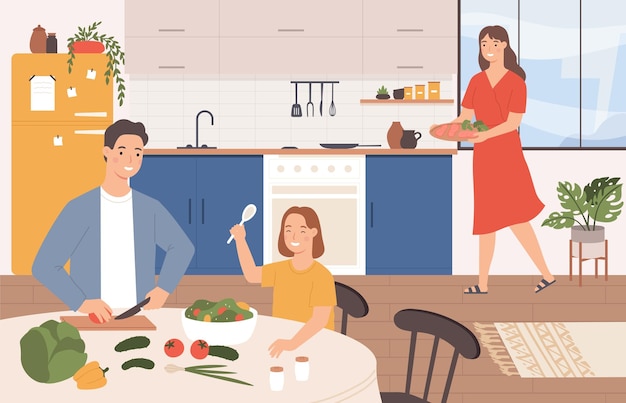This vibrant, slightly cartoonish illustration depicts a warm kitchen scene where a family is preparing a meal. Central to the image, a circular table adorned with a white tablecloth holds an array of vegetables including tomatoes, cucumbers, a yellow bell pepper, cabbage, and green onions. The father, seated with a black knife in his right hand, skillfully chops a tomato on a cutting board, while his young daughter nearby, holding a white wooden spoon, mixes the chopped salad. The table also features other essentials like salt and pepper shakers with orange tops and a white bowl already brimming with prepared salad. 

In the background, the mother, clad in a red summer dress and sandals, strides towards the stove carrying a plate with three raw steaks, ready to be cooked. The kitchen is detailed with blue and white cabinets, a white sink, and white appliances. Directly to the left of the scene stands an orange-yellow refrigerator, adorned with fluttering notes or butterfly-like magnets and topped with two jars and a potted plant with green leaves cascading down. 

Above the scene, kitchen utensils like a spatula, tong, and whisk hang conveniently above the stove. A large blue-tinted window to the right illuminates a lush monstera plant, adding a touch of nature. Below, the carpet on the brown wooden floor enhances the cozy feel of the space, completing this lively and inviting family kitchen tableau.